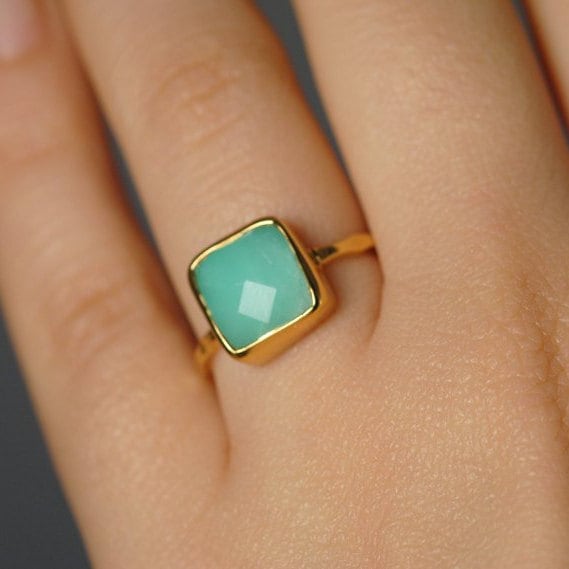This image is a close-up photo focused on a golden ring on the ring finger of a woman's left hand, which has beige or caucasian skin. The ring features a prominent gold band and a large, chunky square centerpiece. The centerpiece is bordered with gold and houses a turquoise or teal gemstone, possibly an opal or turquoise stone, that appears to reflect light. The detailed shot shows only parts of the pinky, ring, and index fingers, highlighting the skin's texture and pores, all set against a gray background.